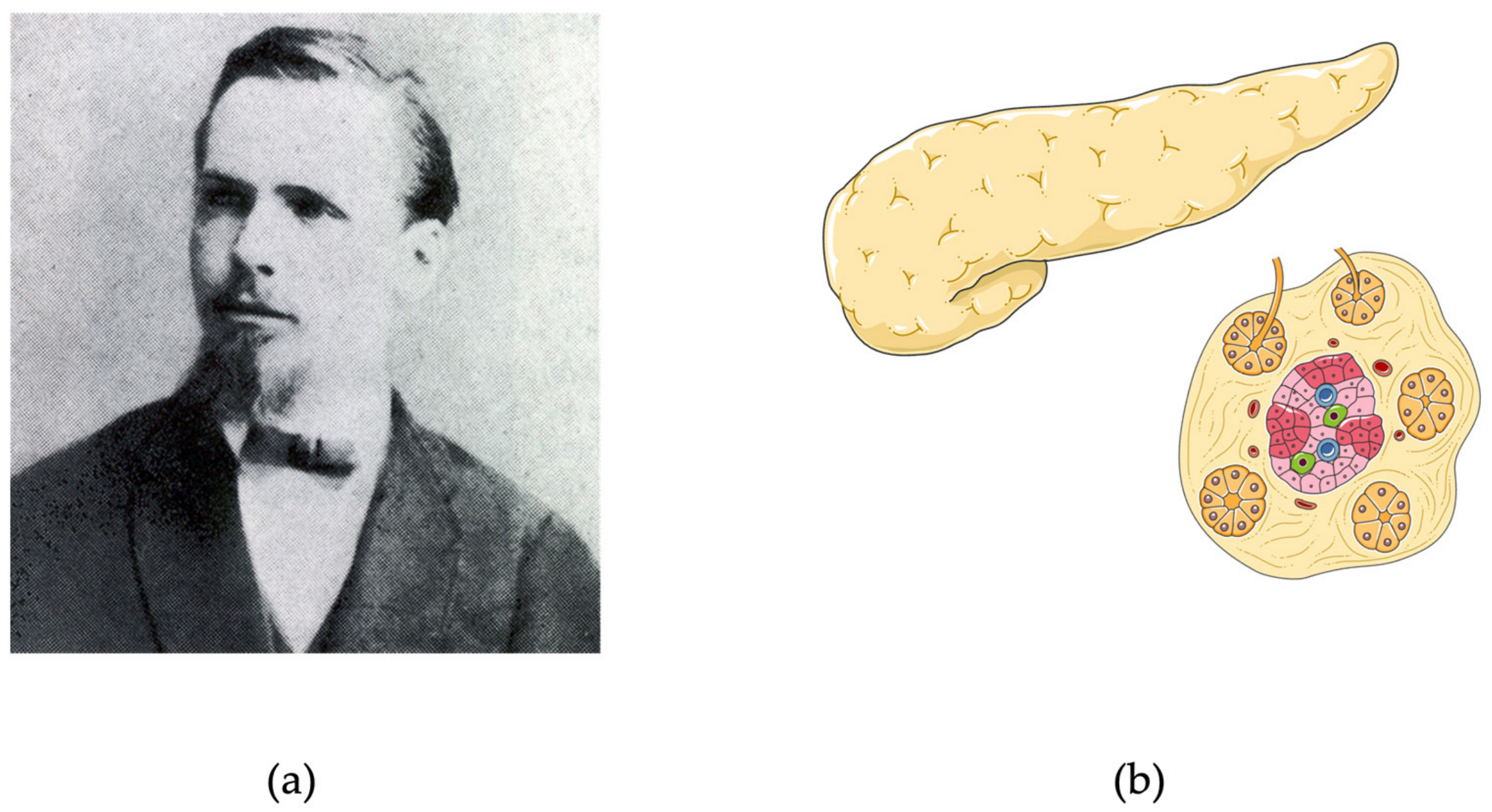The image features two primary illustrations labeled A and B. On the left, labeled A, is a detailed black-and-white portrait of a young man, likely in his thirties. He is dressed in a dark suit jacket and a bow tie with a white shirt underneath. He has a goatee and his hair is parted on the left, combed back neatly, and he's gazing off to his right, away from the camera.

To the right of this portrait, labeled B, is a color illustration resembling a combination of an anatomical and abstract drawing. The upper part depicts a finger-like structure pointing, accompanied by an interior cross-section underneath. This cross-section reveals five circular compartments, each divided into eight slices, reminiscent of a pizza. The circles feature a small dot near their outer edges and lines connecting them to the center. The central section holds a complex, cellular structure with clusters of colors including pink, magenta, blue, green, and red, evoking an abstract representation of internal organs or a biological diagram.